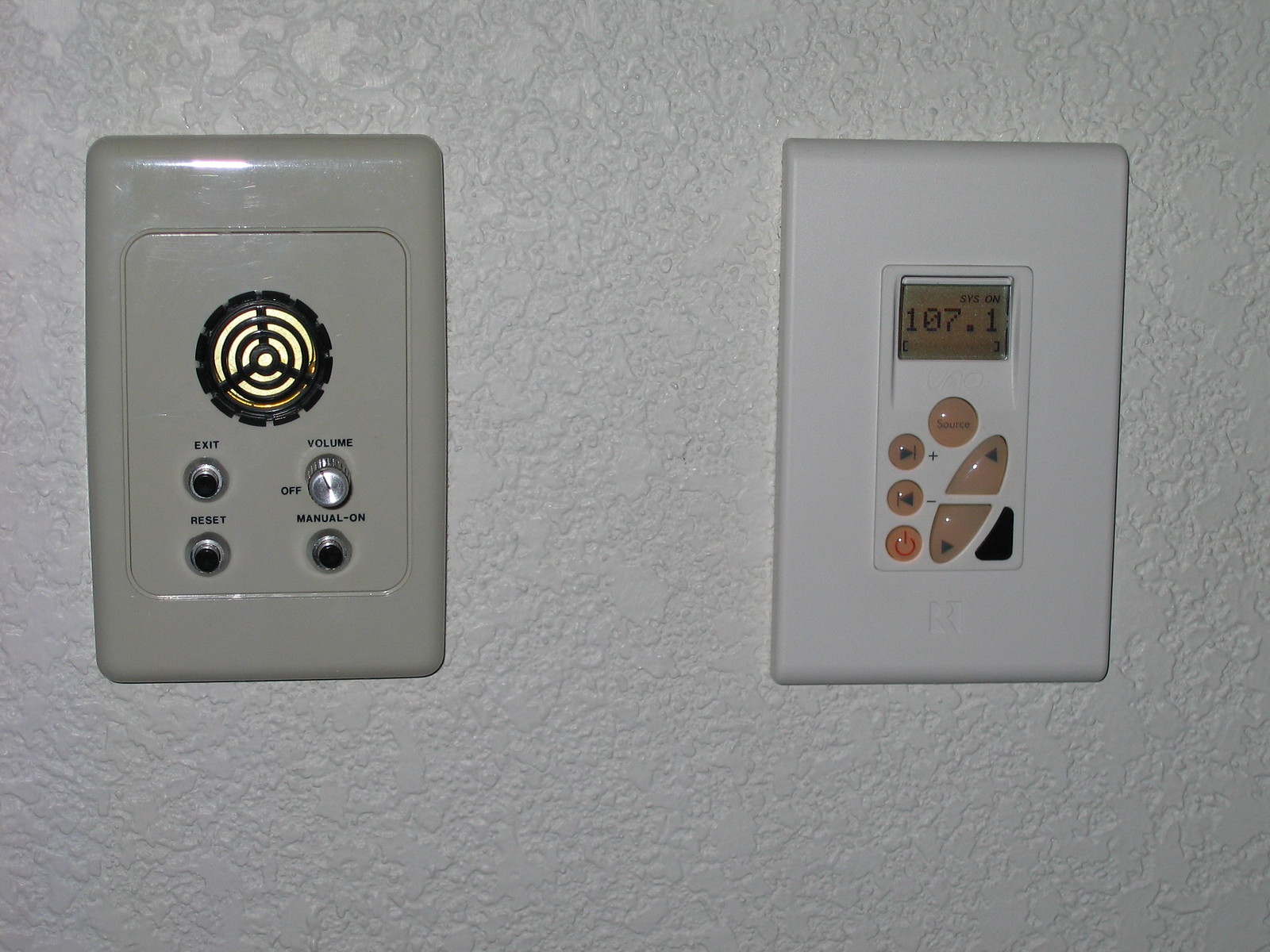The image shows two wall-mounted control panels, positioned side by side. Both panels are rectangular and appear to be used for household functions. 

The panel on the right has a contemporary design with a sleek white frame. It features a small, landscape-oriented digital screen at the top, displaying the number "107.1." Below the screen are multiple round buttons, likely for adjusting various settings, such as tuning or volume control.

The panel on the left is made of a grey plastic material and has a more utilitarian appearance. It is dominated by a central circular knob labeled "Volume," which suggests it is used for audio control. Flanking the knob are four smaller buttons, potentially for additional audio settings or functions.